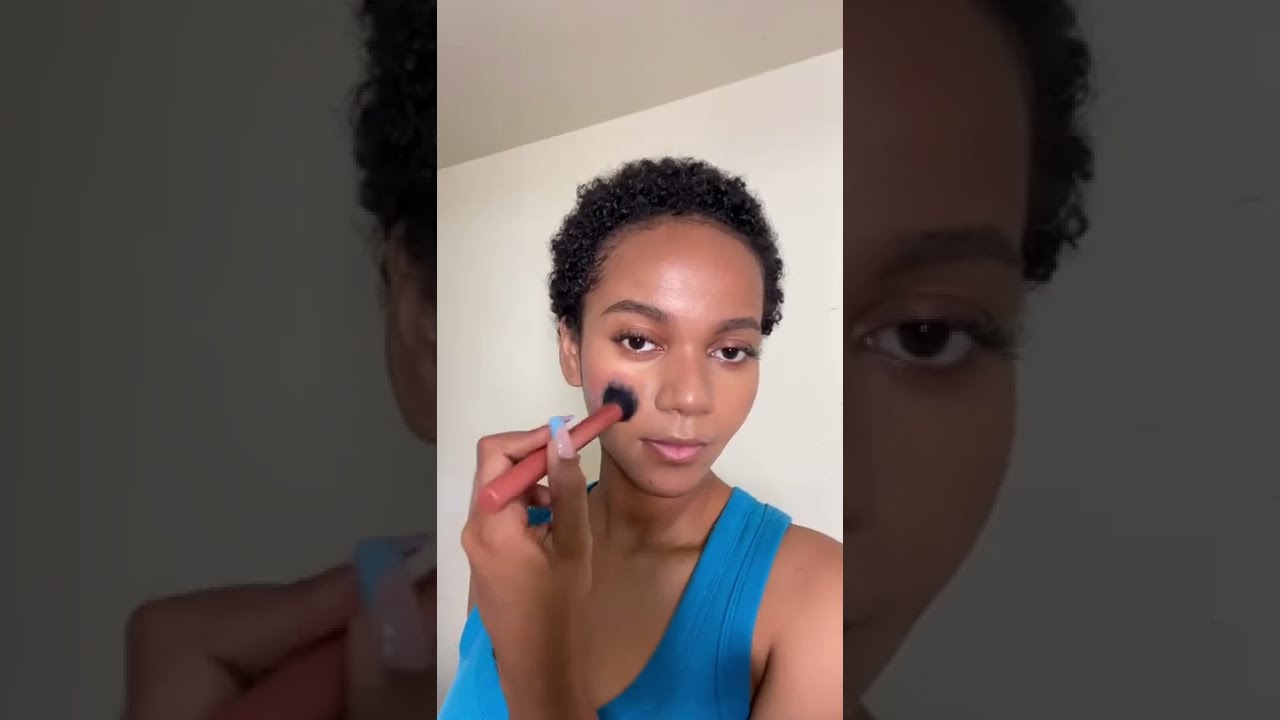This is a wide, three-panel indoor photograph with a central narrow image flanked by two enlarged, darker, and close-up sections of the same image. The central panel, which is the smallest and brightest, features an attractive young black female with light brown skin, short curly black hair, and brown eyes. She is dressed in a blue tank top, with only her shoulders and face visible. The woman is looking directly at the camera while holding a bronzed makeup brush with a long red handle to her cheek, seemingly applying blush. Her nails are painted pink, and the background consists of a simple white wall and ceiling, with a subtle diagonal line marking where the two meet. The left and right panels are blown-up portions of the center image, shaded much darker, adding depth to the composition.